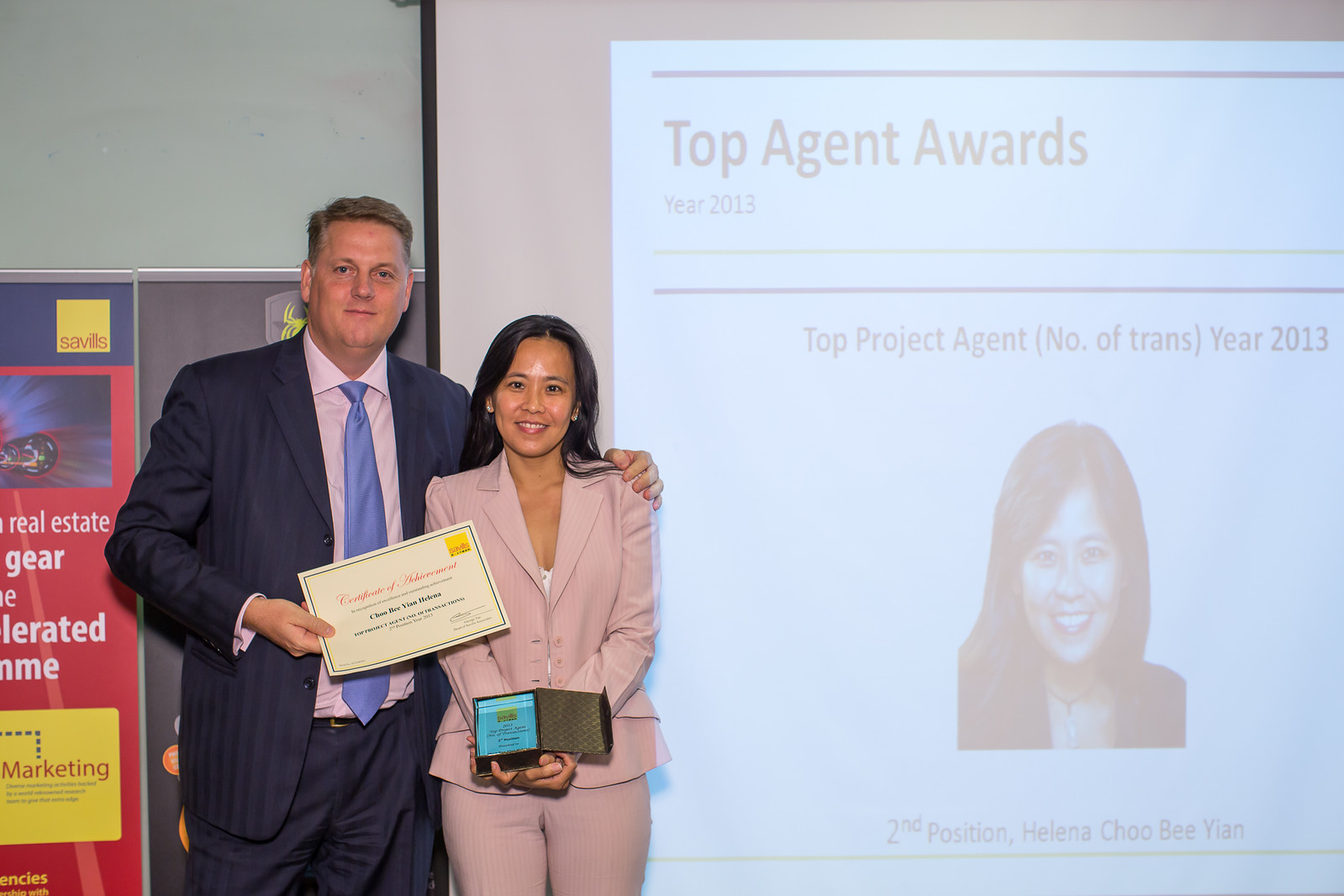In this photo taken during the 2013 Top Agent Awards ceremony, Helena Chu-Bien is being recognized for her second position as the Top Project Agent with the highest number of transactions. Helena, dressed in a pink suit, stands proudly beside her boss who sports a dark blue suit with a light blue tie and a pinkish shirt. The boss is holding a certificate while Helena holds a box in her hand. They are positioned next to a large screen displaying: "Top Agent Awards, Year 2013," which includes her achievement details and a picture of Helena herself. The background also features two banners, one red and one gray, adding to the formal ambiance of the indoor ceremony.